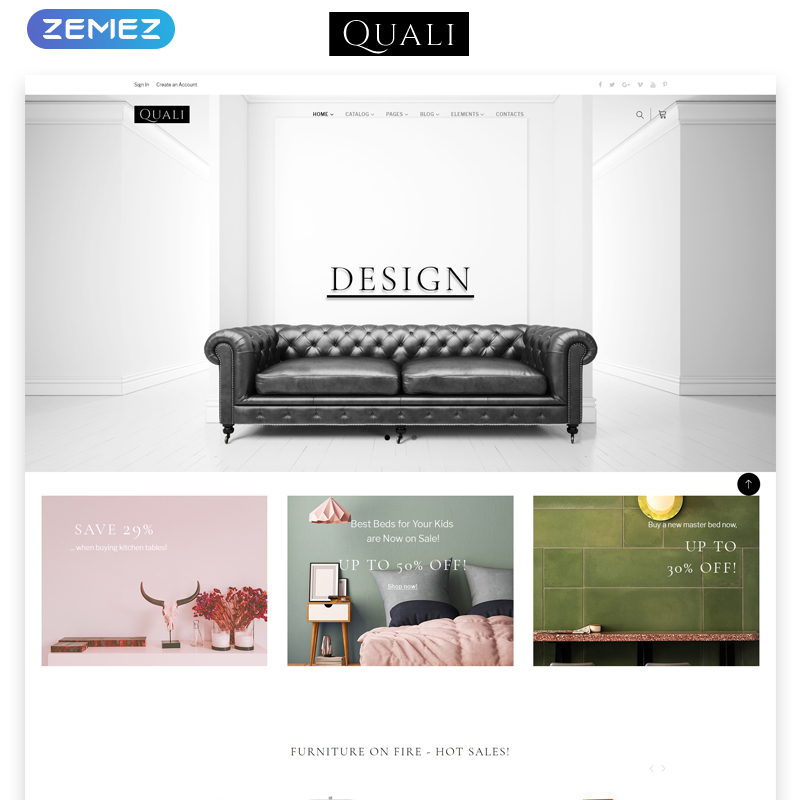The image appears to be a vertical screenshot from a website or web page, possibly an email viewed on a computer or smartphone. The background primarily utilizes the white color of the computer screen. 

At the top left is a blue bar with jagged white letters spelling "Zemez" (Z-E-M-E-Z). In the middle, there is a black box with white text that reads "Quali" (Q-U-A-L-I). A long white strip stretches across the image. On the left side, there are options to "Sign In" or "Create an Account," while on the right side, social media icons are visible. 

Below this, we see a picture of a leather couch with white wood floors and white walls. Above the couch, the word "Design" is underlined. In the upper left of this section, the word "Quali" appears again. Below this, there is a navigation menu with clickable options: "Home" (currently selected), "Catalog," "Pages," "Blog," "Elements," and "Contacts." There's also a search icon, a magnifying glass, and a shopping cart icon within this section.

Further down, there are three promotional squares. 
- The first square has a pink background with various knickknacks and reads, "Save 29% when buying kitchen tables."
- The middle square showcases bedding and pillows, accompanied by the text, "Best beds for your kids are now on sale up to 50% off. Shop Now."
- The last square, with a green tile background resembling a countertop, states, "Buy a new master bed now up to 30% off."

At the bottom of the image, bold black capital letters proclaim, "FURNITURE ON FIRE HOT SALES."